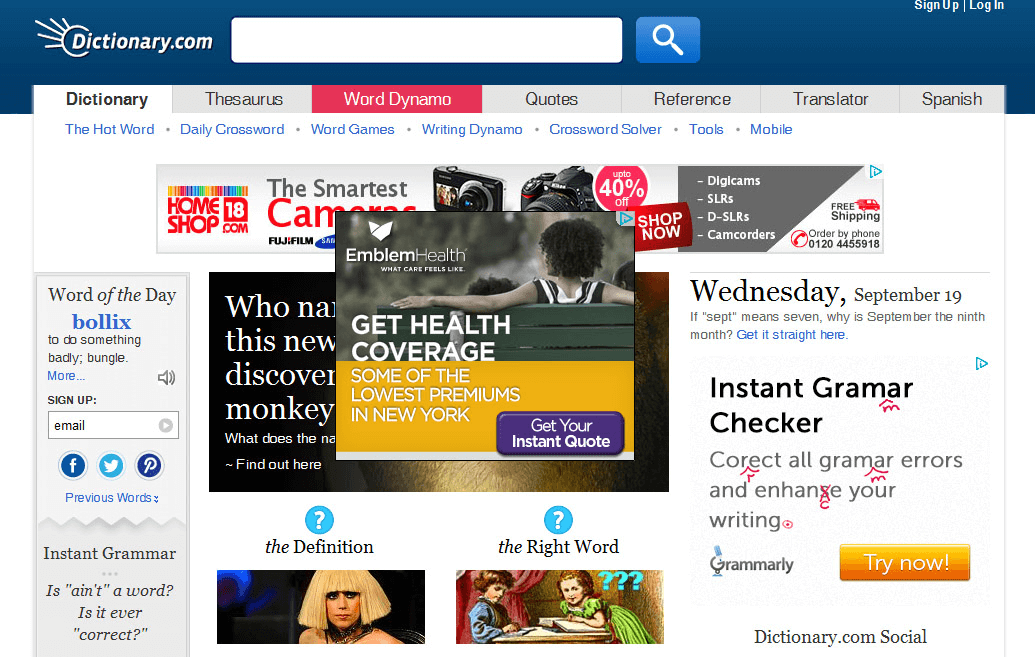This image is a screenshot of the Dictionary.com website. The top of the page features a blue border with the Dictionary.com logo in the upper left corner. The logo consists of the word "Dictionary" in white, followed by ".com" and is encircled by a series of five radial lines emanating from the back.

Below the logo is a white search bar with a blue search button to its right. Adjacent to this search bar is a section for users to sign up or log in to their accounts. 

Directly under the search bar and login area, a navigation banner offers various options, including 'Dictionary,' 'Thesaurus,' 'Word Dynamo,' 'Quotes,' 'Reference,' 'Translator,' and 'Spanish.' It appears that the user is currently on the 'Dictionary' tab.

The screen is cluttered with several pop-up ads. Central among these pop-ups is a square ad framed in gray. The ad features an image of an individual, presumably female and African-American, sitting on a bench with a small child. The adult's arm is draped over the back of the bench, with only their black hair visible over the top.

In the upper left corner of the ad, the text "EmblemHealth" is displayed. Below the bench, on the left side of the ad, the text reads "Get health coverage." At the bottom of this pop-up is a yellow rectangular section stating, "Some of the lowest premiums in New York." To the right of this text is a purple rectangular button labeled "Get your instant quote."